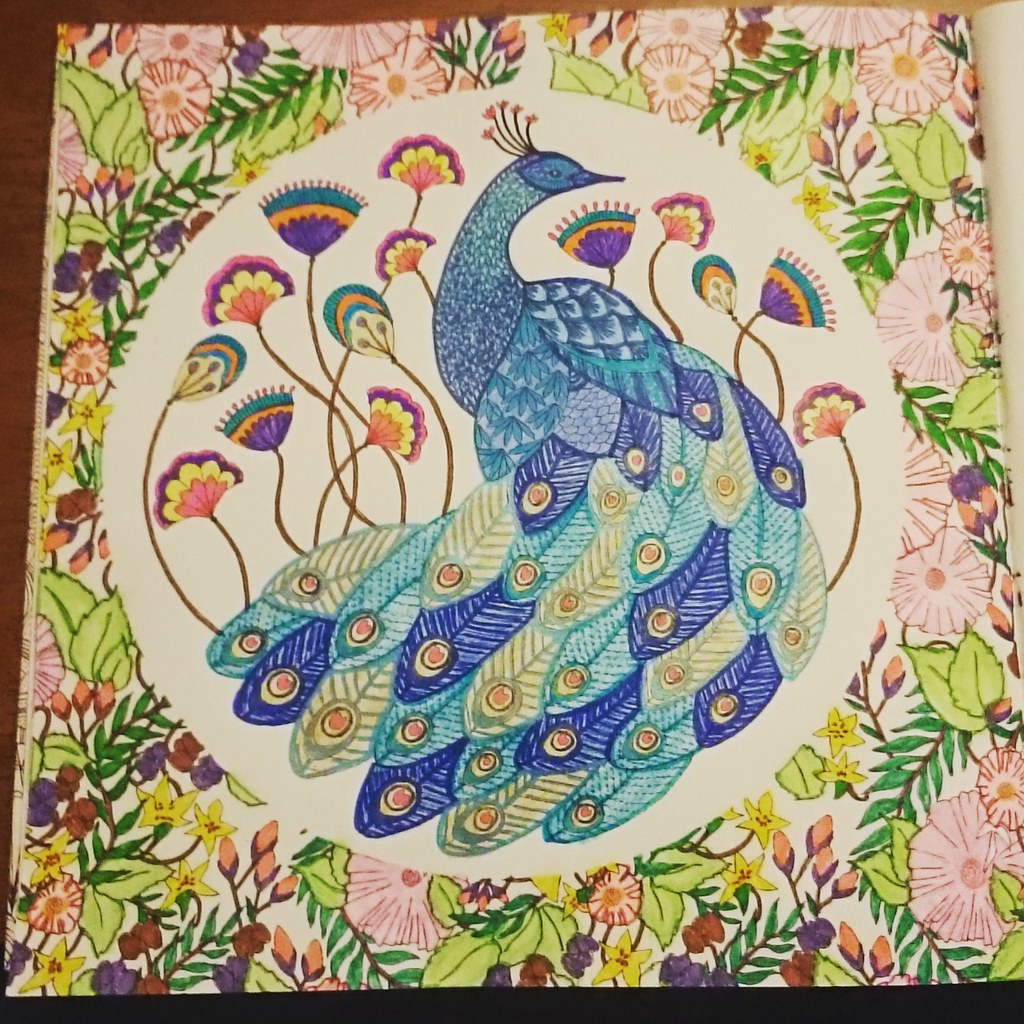The detailed painting, sketched with pencils and colored using colored pencils and markers, features a striking blue peacock as its central focus. This peacock, depicted within a white circular background, exhibits an intricate combination of dark and light blue tones, complemented by yellow and green hues on its feathers. The peacock’s head showcases five orange-topped strands, while its eyes and beak are emphasized with dark triangular markings. Surrounding the majestic bird is a collage of vibrant feathers, each varying in shades of yellow, light blue, and dark blue with circular orange tips.

Embracing the circular frame, an array of flowers and leaves bloom with splendor. These flowers, in diverse shades of pink, purple, green, and yellow, provide a vivid contrast against the peacock's striking colors. Some flowers emerge directly from the peacock’s body, extending outward, while others encircle the bird, further enhancing the composition's rich detail. The outer edges of the image transition from a dark orange to a brown hue, adding depth and warmth to the overall aesthetic. This intricately designed and colorfully vivid picture showcases the beauty of both the peacock and the surrounding flora in a harmonious blend.